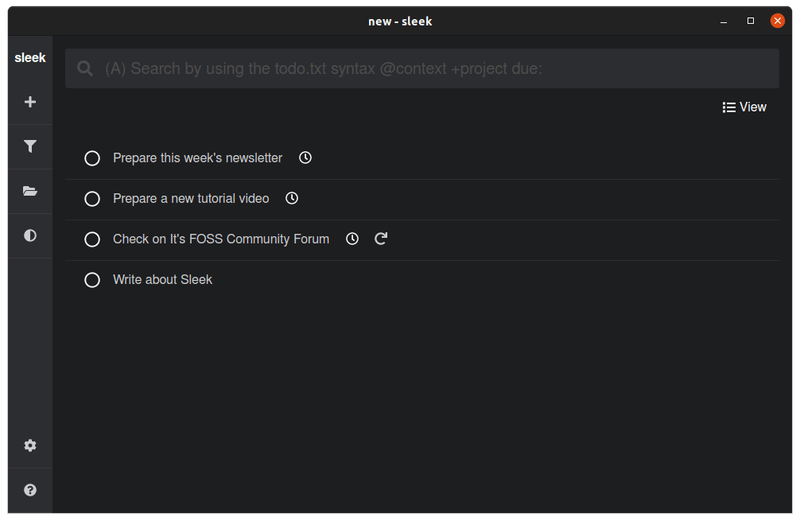This detailed caption serves to accurately describe every element of the image:

---

The image is a dark mode screenshot captured on a PC or tablet screen interface. At the very top, the words "new-sleek" appear prominently in white font. On the left side of the screen, a vertical toolbar features several icons arranged from top to bottom. These include a 'sleek' tab, a 'plus sign (+)', and an 'internet' icon, though its purpose is uncertain. Following these are a 'file' icon, a 'dark mode/light mode' toggle icon, a 'settings' icon, and a 'fax' icon.

In the central area of the screen, a search bar is visible with the prompt, "Search by using the total text." Below this prompt, a list of tasks or search suggestions is displayed, consisting of:
- "add context"
- "project due"
- "prepare this week's newsletter"
- "prepare a new tutorial video"
- "check the FOSS community forum"
- "write about sleek"

On the right side of the screen, there are additional control icons. These include an icon to close the current screen (distinct from an exit icon meant to close the application), an icon of a large square, and an exit screen icon which likely serves to close the application or window entirely.

---

This caption provides a comprehensive and clear description of the image, covering all the visual elements mentioned.